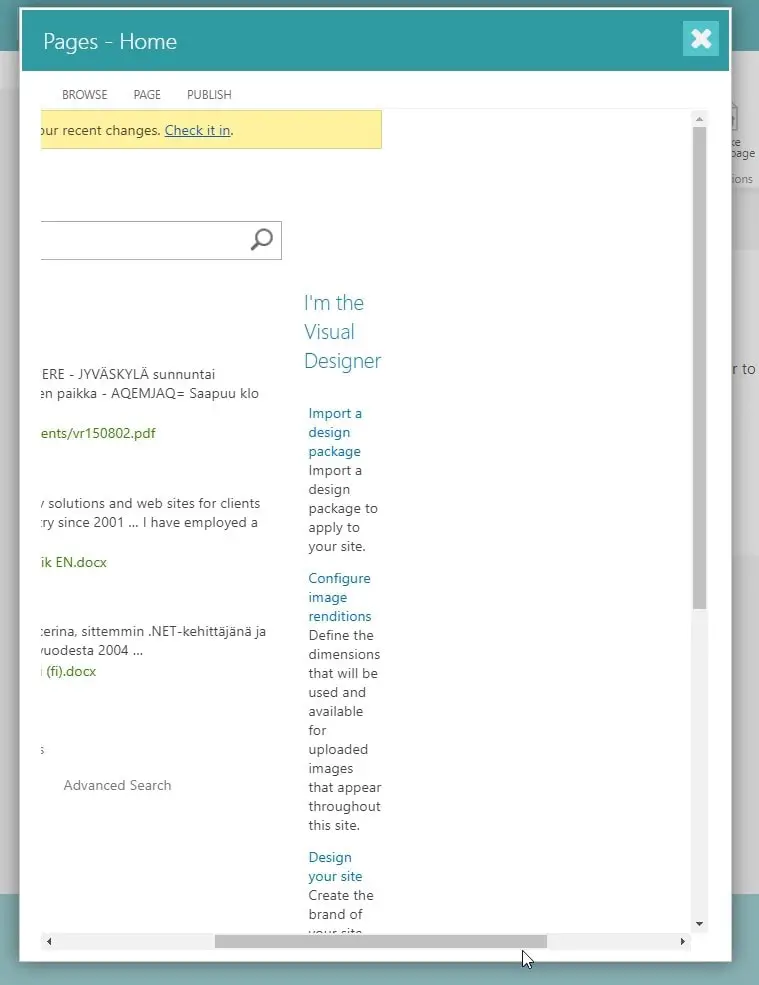The image displays an online page featuring a user interface with multiple interactive elements. At the top, a green banner spans across the page, with an "X" icon for closing the banner located in the upper right corner. On the left-hand side, the text "Pages - Home" is prominently displayed. Below the green banner, a white border contains several navigational titles aligned horizontally: "Browse," "Page," and "Publish."

Immediately beneath this, a yellow banner is partially visible, indicating that the screen has been scrolled to the right. From what is visible, the banner shows the text "Recent Changes" and includes a hyperlink labeled "Check it in." 

Further down, a search bar allows users to enter search criteria. The results include multiple documents, each identified by their respective file extensions such as PDF and DOCX. The right pane of the window appears to provide additional details about the selected documents, listing various functions and features like "Visual Debugger," "Import a Design Document," "Configure Image Renditions," and "Design Your Own Site." 

Additionally, the scroll bar's position indicates that the left portion of the screen is partially obscured, limiting the view of certain elements on the interface.